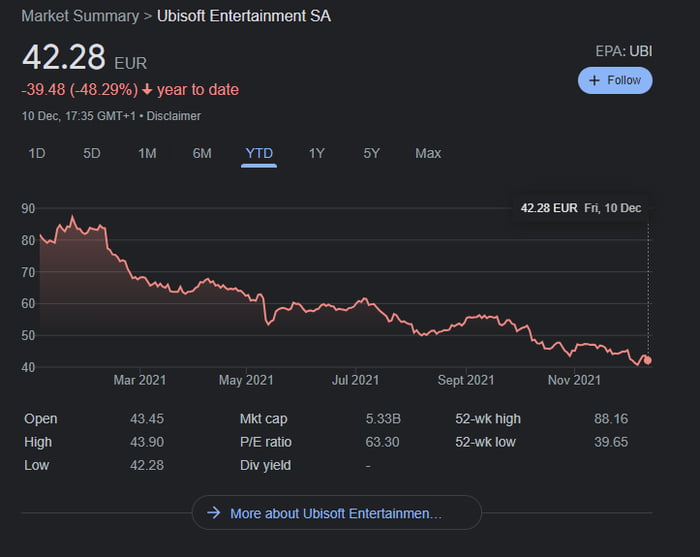**Caption:**

A detailed market summary for Ubisoft Entertainment SA is displayed on a stock tracker interface against a black background with white lettering. The current stock price is €42.20, labeled alongside the ticker symbol EPA:UBI and a blue plus mark with a follow button. Underneath, the stock shows a year-to-date loss of -€39.48 or -48.29%. The data is time-stamped 10th December, 17:35 GMT+1. 

Various time range options are visible at the top, including 1 Day, 5 Day, 1 Month, 6 Month, Year-to-Date, 1 Year, 5 Year, and Max, with Year-to-Date currently selected. The red graph indicates a significant decline from a value slightly over €90 in March 2021 to the current price of €42 in November. 

At the bottom, additional specifics are provided:
- Open: €43.45
- High: €43.90
- Low: €42.20
- Market Cap: €5.33 billion
- P/E Ratio: 63.30
- Dividend Yield: N/A
- 52-Week High: €82.15
- 52-Week Low: €39.65

A blue button to the right invites users to learn more about Ubisoft Entertainment.